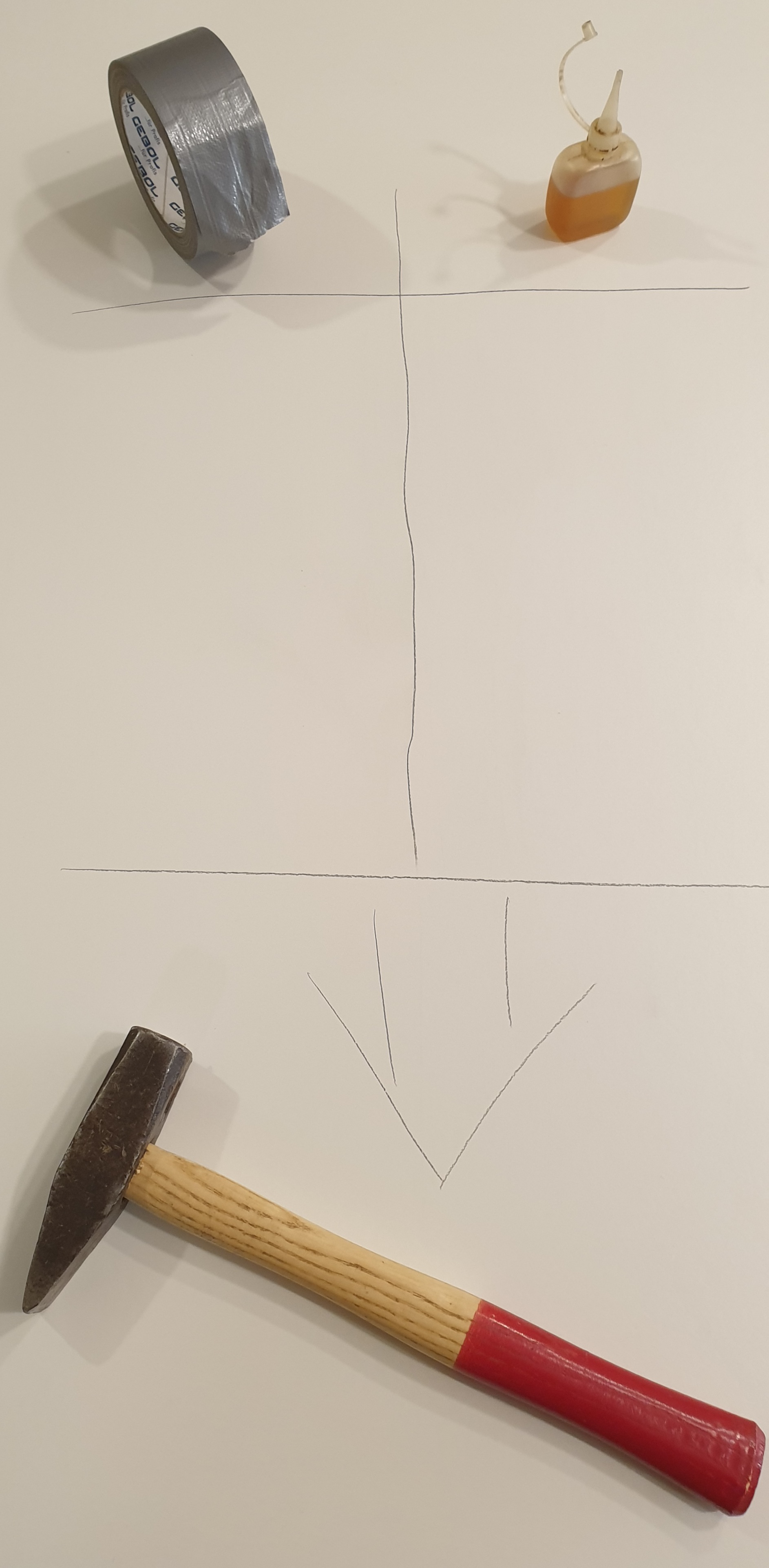The image portrays a meticulously arranged scene featuring a few tools and a marked surface. On the top left, a roll of duct tape is positioned vertically, next to a light brown bottle of glue. Beneath these items, on a clean white floor, there are precise lines drawn, likely with a pencil or pen. One line runs horizontally under the duct tape and glue, intersected by a vertical line that extends downward to another horizontal line. An arrow has been sketched on the floor, directing attention to a hammer located at the bottom of the image. The hammer features a metal head with one end sharply pointed and the other end flat, complemented by a wooden handle that transitions to a red color at its base. The scene is clearly and deliberately composed, drawing focus to the tools and their arrangement.